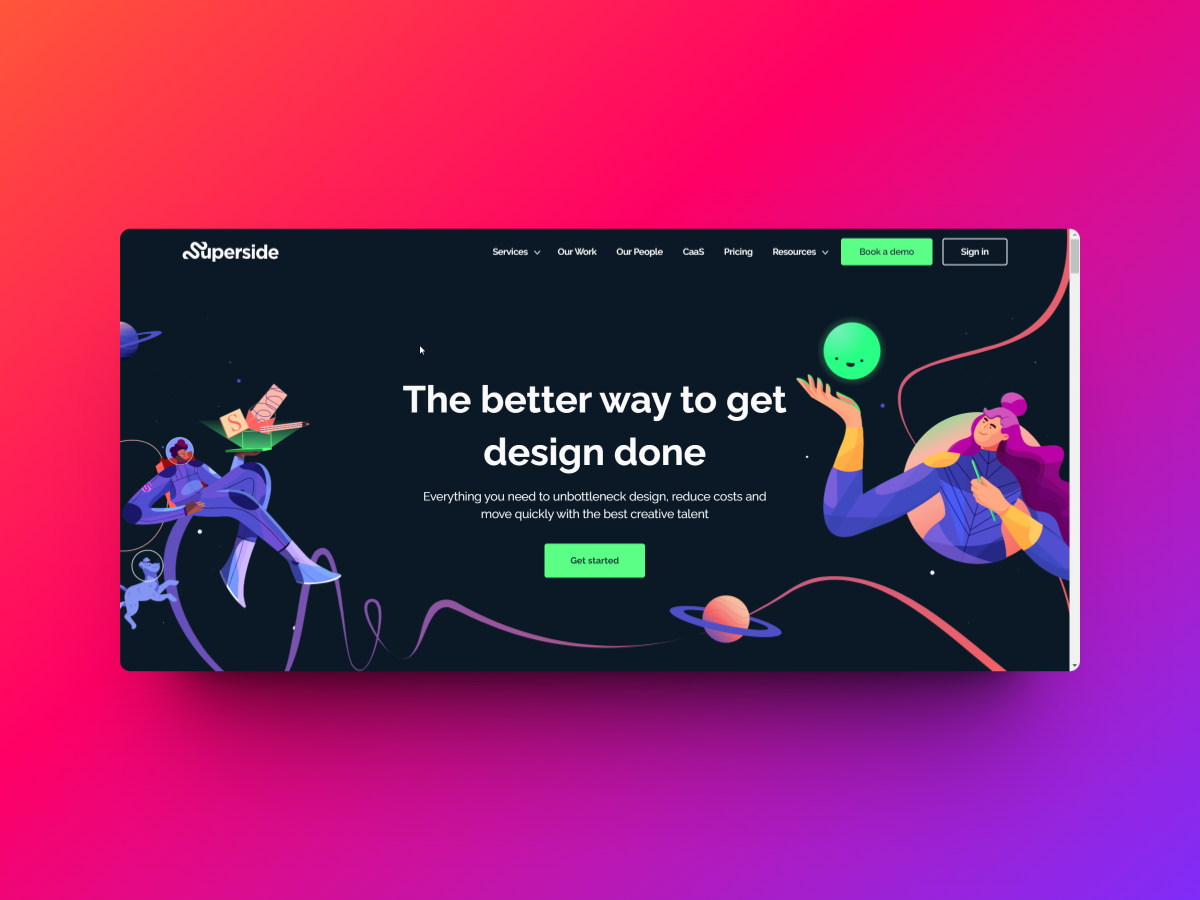The image is a wide horizontal rectangle filled with vibrant gradients. The background features a gradient that transitions from orange in the upper left corner, to coral, hot pink, light purple, and finally dark purple as you move across to the bottom right corner. This purple color deepens along the bottom third of the image before shifting back to pink and coral as it approaches the bottom left corner.

Overlaid onto this colorful background is a smaller, horizontal, black rectangle. In the top left corner of this black rectangle, "Super Side" is written in white font. Below this, white-font-labeled columns appear with pull-down menus, including labels such as "Services," "Our Work," "Our People," and "Resources," though a couple are unreadable. Adjacent to these is a green button labeled "Book a Demo" in black font, followed by a "Sign In" button in white font.

Centered on this black rectangle is a large, bold, white-font slogan: "The Better Way to Get Design Done." Beneath this slogan, a smaller white font reads, "Everything you need to unbottleneck design, reduce costs, and move quickly with the best creative talent." Below this text, a green rectangular button with black text reads, "Get Started."

In the detailed illustration, a purple planet resembling Saturn with a ring is positioned towards the top left. Below the planet is an astronaut reclining, holding a piece of paper and other items in their left hand, with a small dog sitting nearby. On the right side of the image, a woman with long pink hair is depicted. She has her right hand raised, holding a green circle with a face above her, almost like a bowling ball, while clutching another item in her other hand. Another ringed planet is visible slightly right of the middle of the image.